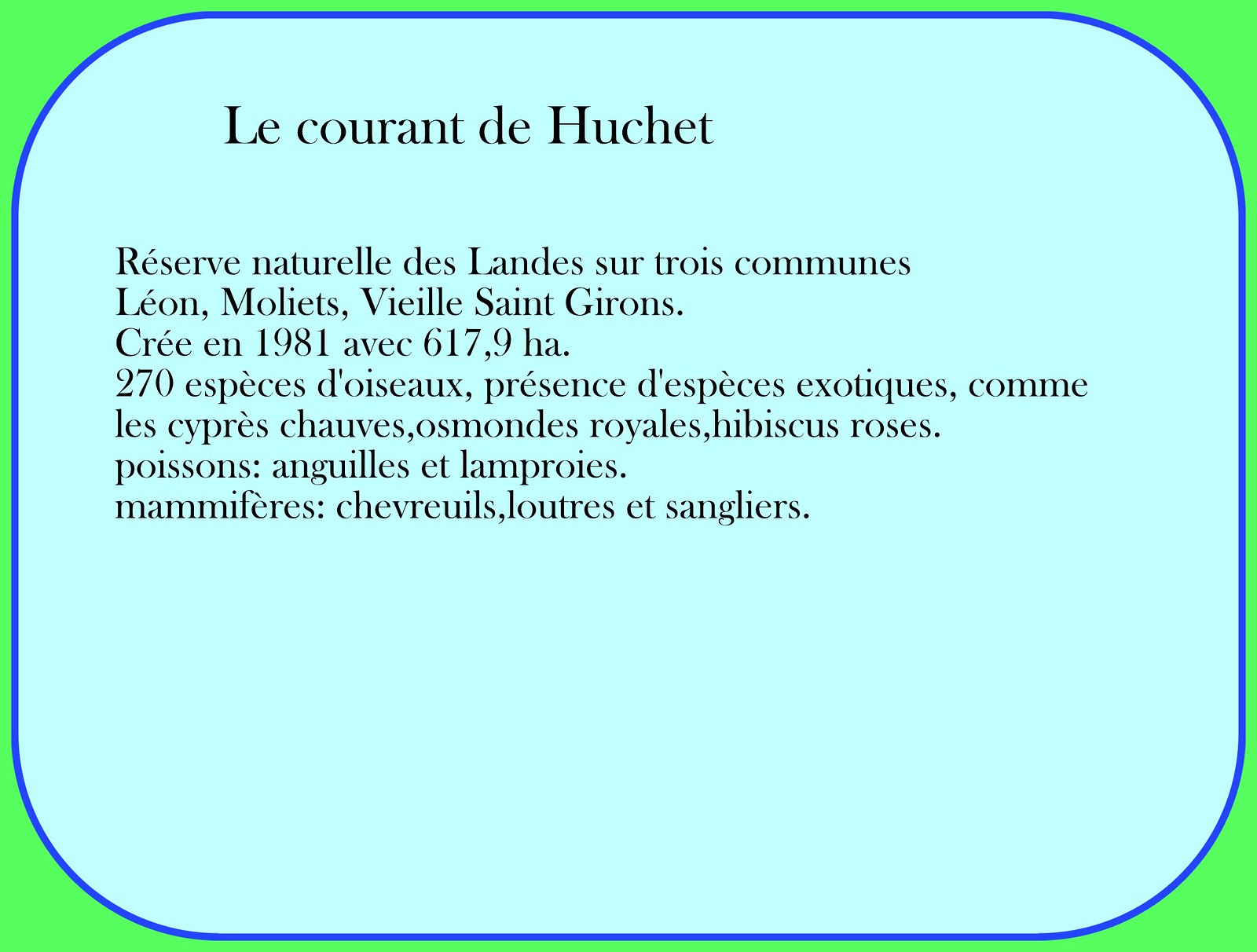This PowerPoint slide features a vibrant green background, prominently contrasted by a blue section below the text area. Enhancing the aesthetic appeal, a darker blue border frames this blue background section. Notably, the blue section includes elegantly curved edges on all four corners, adding a sophisticated touch to the slide design.

The text, which appears to be in French or another Romance language, includes a bold title at the top: "LE COURANT DE HUCHET." Beneath this title, approximately seven lines of text occupy the upper half of the slide, suggesting that the content is brief yet informative. The exact details of the text remain unclear due to language barriers. This slide likely serves as an introduction or overview, given the positioning and prominence of the title.